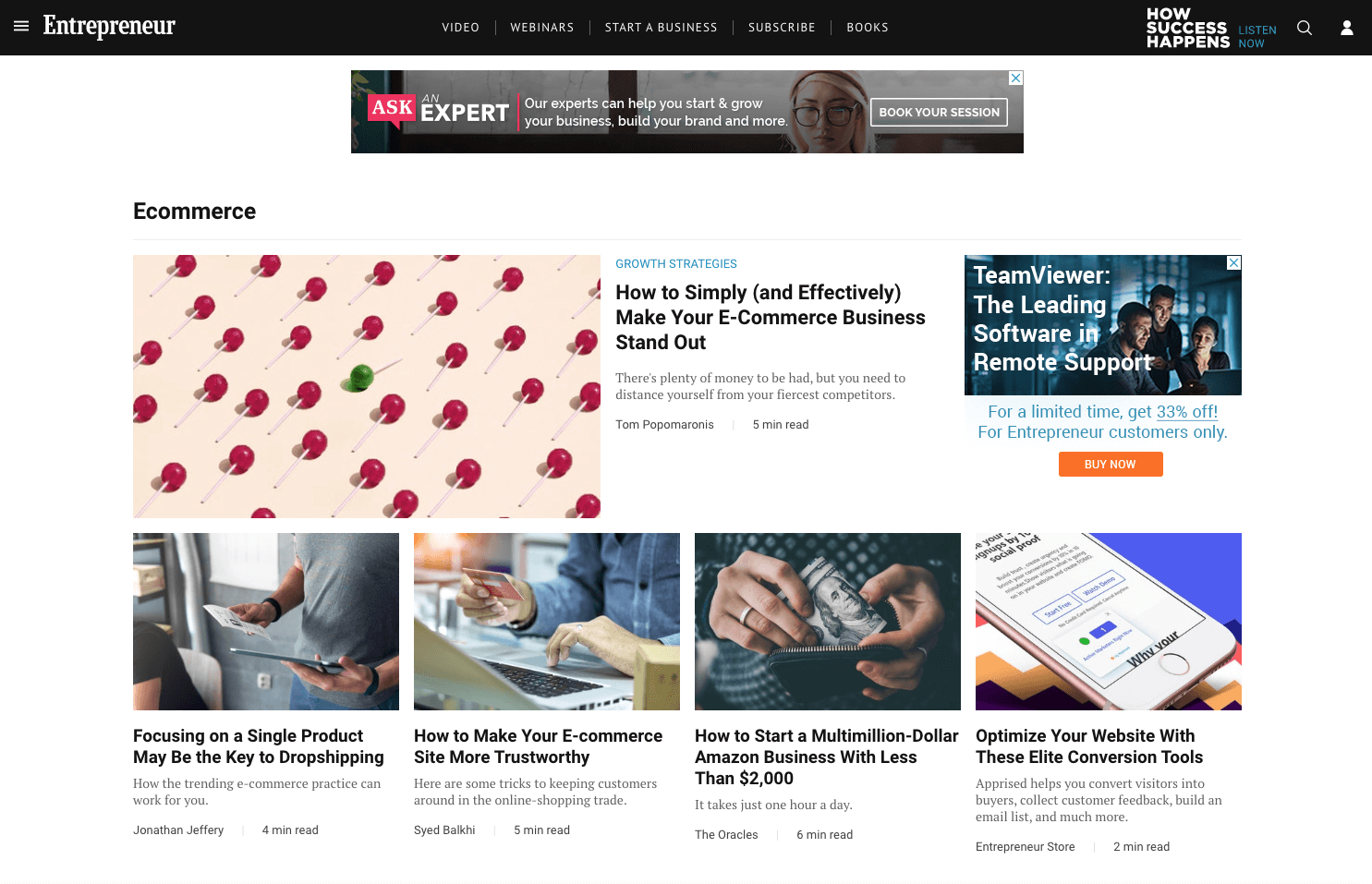**Web Page Description: Entrepreneur Platform Overview**

The webpage features a clean design with a predominantly white background. At the top, there's a black border header displaying the word "Entrepreneur." Below this header, there is a small and light text presenting five key points of information in a list format.

On the right side of the page, a section is highlighted with the phrase "How Success Happens," accompanied by icons of a magnifying glass and a profile silhouette. Adjacent to these elements, it reads "Listen Now."

The next segment of the page is a black block prominently featuring the word "ASK" in red, followed by "AN EXPERT" in white text. Underneath, smaller text states, "Our experts can help you start and grow your business, build your brand, and more." This section also includes a photograph of a young woman with blonde hair and glasses, alongside a call-to-action button in a separate rectangle that says "Book Your Session."

Continuing down the page, there is a structured layout of informational content. It includes a grid comprised of three rectangular blocks on the top row and four on the bottom row, all collectively forming one large rectangular section. 

- The first block features an article titled "How to Simply and (Effectively) Make Your E-Commerce Business Stand Out," illustrated with an image of several red lollipops against a pink background, with one distinct green lollipop.
- The second block promotes "TeamViewer: The Leading Software in Remote Support," highlighting an exclusive offer of 33% off for Entrepreneur customers. This block includes an orange rectangle with the text "Buy Now."

The bottom row comprises four additional rectangular blocks providing further insights and tips on starting a business.

Overall, the webpage is visually organized to guide users through an array of resources and services aimed at entrepreneurs.